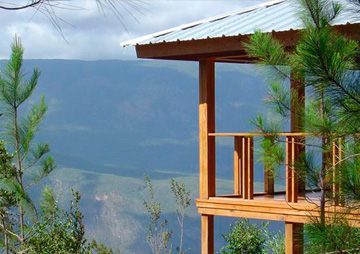In this image, captured from a high vantage point, a panoramic view unfolds. On the right-hand side, vibrant green leaves extend from tree branches, partially obstructing a modest wooden house. The house features a light brown wooden railing and a white roof, resembling a quaint structure ideal for sightseeing. To the left, a cluster of trees frames the scene. In the distance, a hazy, grayish landscape emerges, indicative of the long-distance view, with rolling hills forming a gentle backdrop. Above, a gray sky, streaked with clouds, crowns the horizon. The overall composition showcases a serene and picturesque setting, blending natural elements with a touch of architecture.